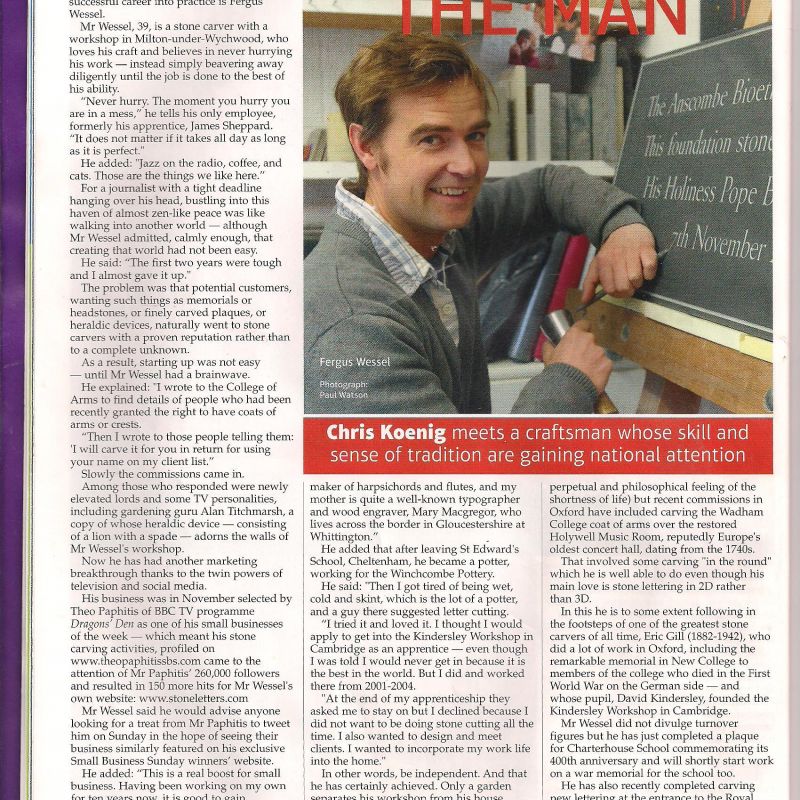The image is a clear screenshot of a possibly published medium, either a newspaper article or a section from a textbook. It features a photograph in the top right corner of a man dressed in a grey sweater layered over a button-up plaid shirt. He has short brown hair and is depicted leaning against a piece of stone, seemingly in the process of carving it. Below this image, a prominent red box contains the text: "Chris Koenig meets a craftsman whose skill and sense of tradition are gaining national attention." The left side of the page, stretching from the top to the bottom, and then continuing in two columns directly beneath the red banner, is densely packed with paragraphs. These texts appear to detail the work and life of the featured carver, highlighting his craftsmanship and the traditional aspects of his skills that are garnering national recognition.